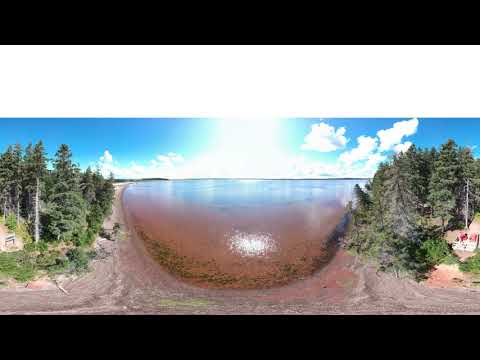This is a detailed 360-degree photograph of a basin-like lake, surrounded by trees and land. In the foreground, the lake appears brown and green due to the murky water mixing with sand. As the water extends toward the background, close to the horizon, it becomes a more typical blue. The sky above is a clear blue, dotted with soft white clouds and a very bright sun positioned centrally in the image. On the left side, there is a light-colored, reverse L-shaped road beside a dense cluster of trees, which predominantly have foliage at the top, with some showcasing long white trunks. To the right, the trees are generally triangular-shaped with lush leaves, but a few have visible trunks. Notably, there's a little white board with two red objects resting on it. Additionally, power lines can be seen on both the left and right sides of the image. At the top of the image is a horizontal white strip, and two horizontal black strips run across the bottom.